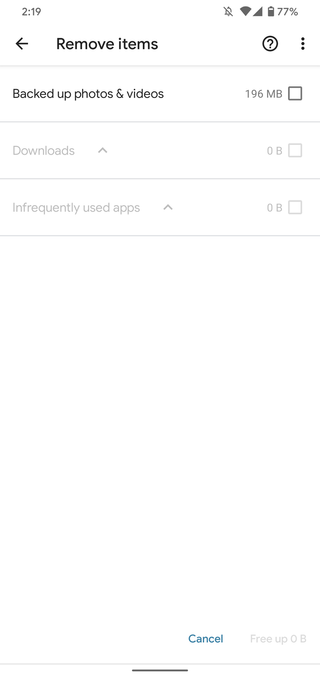This screen capture showcases a smartphone interface of an app with options to remove items. In the top-right corner, the battery level is at 77%, with icons indicating active Wi-Fi and cellular connections, while notifications are turned off. The time displayed in the top-left corner is 2:19. The main section is headed by the title "Remove Items," accompanied by a left-pointing arrow, a help icon (circle with a question mark), and a three-dot menu indicating additional options.

Below the title, three removable item categories are listed:

1. "Back up photos and videos" (196 MB) with an associated checkbox.
2. "Downloads" with an upward arrow and a size of 0B, alongside a checkbox.
3. "Infrequently used apps" with an upward arrow and a size of 0B, also with a checkbox.

At the bottom of the screen, there is a blue "Cancel" button next to a grayed-out "Free up 0B" button. Additionally, a small thin black line is visible at the bottom center, which may represent the sound bar or another interface element.